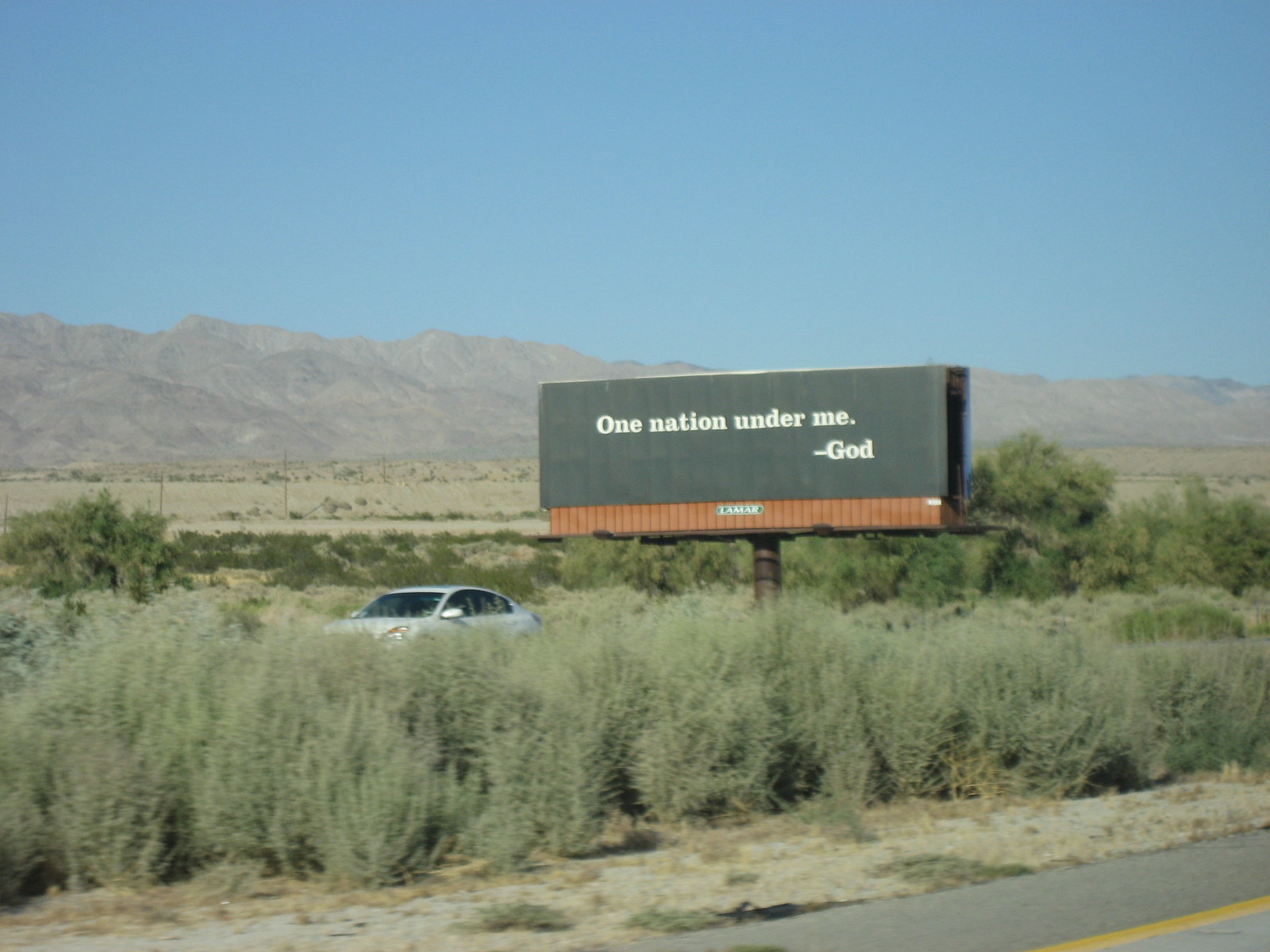In this image, taken from the side of a highway, the bottom right corner reveals a yellow lane line marking the road boundary. The scene features a median densely populated with tall, sage-green bushes, reminiscent of desert vegetation. Through these thick bushes, a white or light silver van is visible, although mostly obscured except for its top part. Further behind the vehicle, a solitary black billboard dominates the center of the image, bearing the white text "One Nation Under Me" with the word "God" beneath it, implying a divine signature. The billboard is mounted on a typical brown, circular post and has a brown frame at its base. In the background, scattered trees give way to a sweeping vista of desert terrain, culminating in a range of imposing mountains that stretch across the image. The sky overhead is a clear, vibrant blue, suggesting this photo was taken during daylight hours. The overall scene evokes the arid landscapes of inland Southern California, Arizona, or New Mexico.